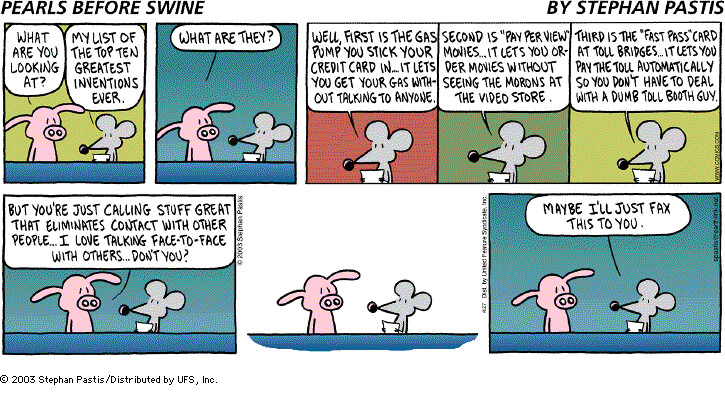This is a detailed cartoon strip from the comic series "Pearls Before Swine" by Stephan Pastis. The cartoon is composed of five squares on top and three larger rectangles underneath, all with a mix of colored backgrounds — yellow, blue, white, and red. The text is written in black, with dialogue in bubble writing.

The cartoon features a pig, who is pink, and a mouse, who is gray with a black nose. In the first row of panels, the pig asks, "What are you looking at?" The mouse replies, "My list of the top 10 greatest inventions ever." The pig follows up with, "What are they?"

In the three subsequent larger rectangles, the mouse elaborates on the first three items on his list:
1. "First is the gas pump you stick your credit card in. It lets you get gas without talking to anyone."
2. "Second is a pay-per-view movie. It lets you order movies without seeing the morons at the video store."
3. "Third is the fast pass card at toll bridges. It lets you pay the tolls automatically so you don't have to deal with a dumb toll booth guy."

In the final part at the bottom of the strip, the pig retorts, "But are you just calling stuff great that eliminates contact with other people? I love talking face-to-face with others, don't you?" After a moment of silence, the mouse concludes with, "Maybe I'll just fax this to you." The characters appear positioned facing each other, although it's unclear if they are standing or sitting. The cartoon's style mirrors typical newspaper or magazine comic strips.